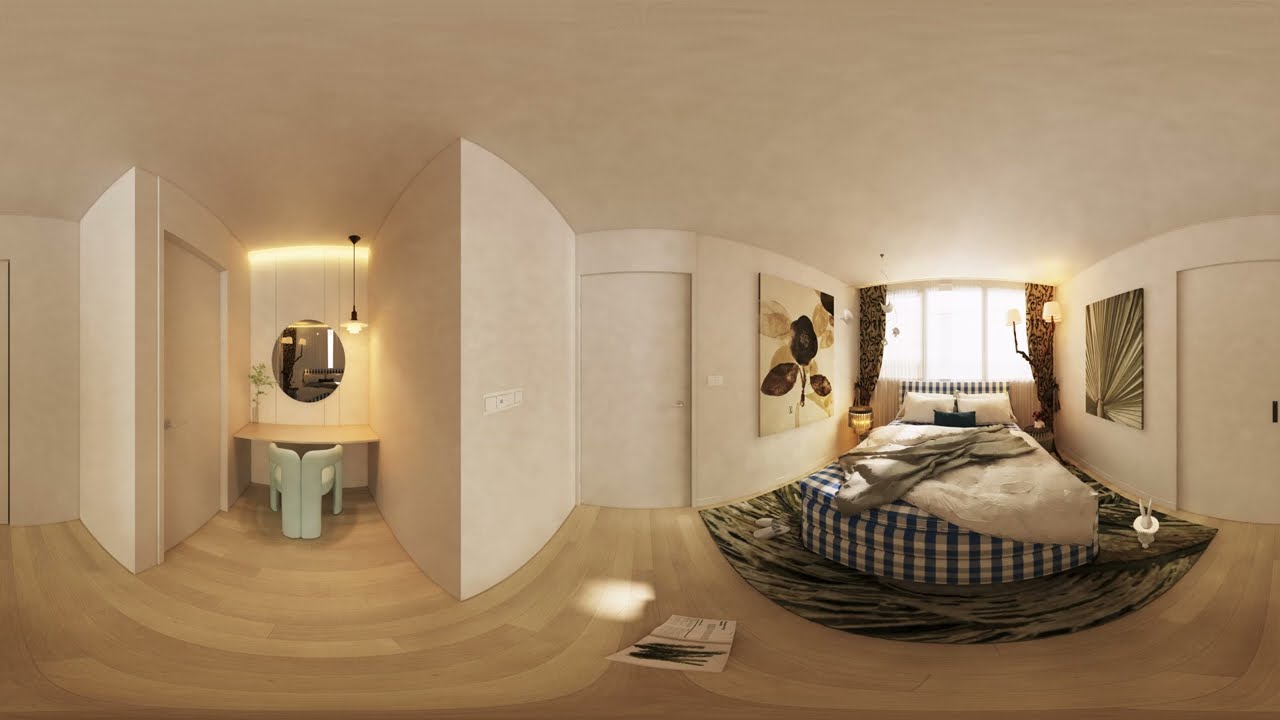This horizontally-aligned rectangular image, taken indoors during the daytime, presents a spacious room without a wall separating two main areas. The ceiling is a light tan or beige color, matching the walls. The flooring throughout is light brown wood paneling. 

On the left side of the image, there are two walls forming a cubby area that houses a small rectangular desk with a light green chair. Above the desk, a circular mirror is mounted, accompanied by a hanging light fixture from the ceiling. Moving toward the center-left, a white closed door appears, followed by a shelf in the seating area for placing items.

Transitioning to the right side of the room, the middle section features another white closed door and a centered window composed of three panes, with gold and black drapes on either side. Against this back wall under the window is a bed adorned with blue, gray, and white checkered bedding, a couple of white pillows, and a gray fabric throw casually draped over the bed. Below the bed appears a rug with black and tan colors.

Framing the bed, two large square canvas-like images in shades of gold, black, and brown decorate the walls, one next to the bed and another by the second door further right. The photo captures the serene and organized setting of a master bedroom, with a balanced mix of light brown, white, blue, gray, gold, and black hues.